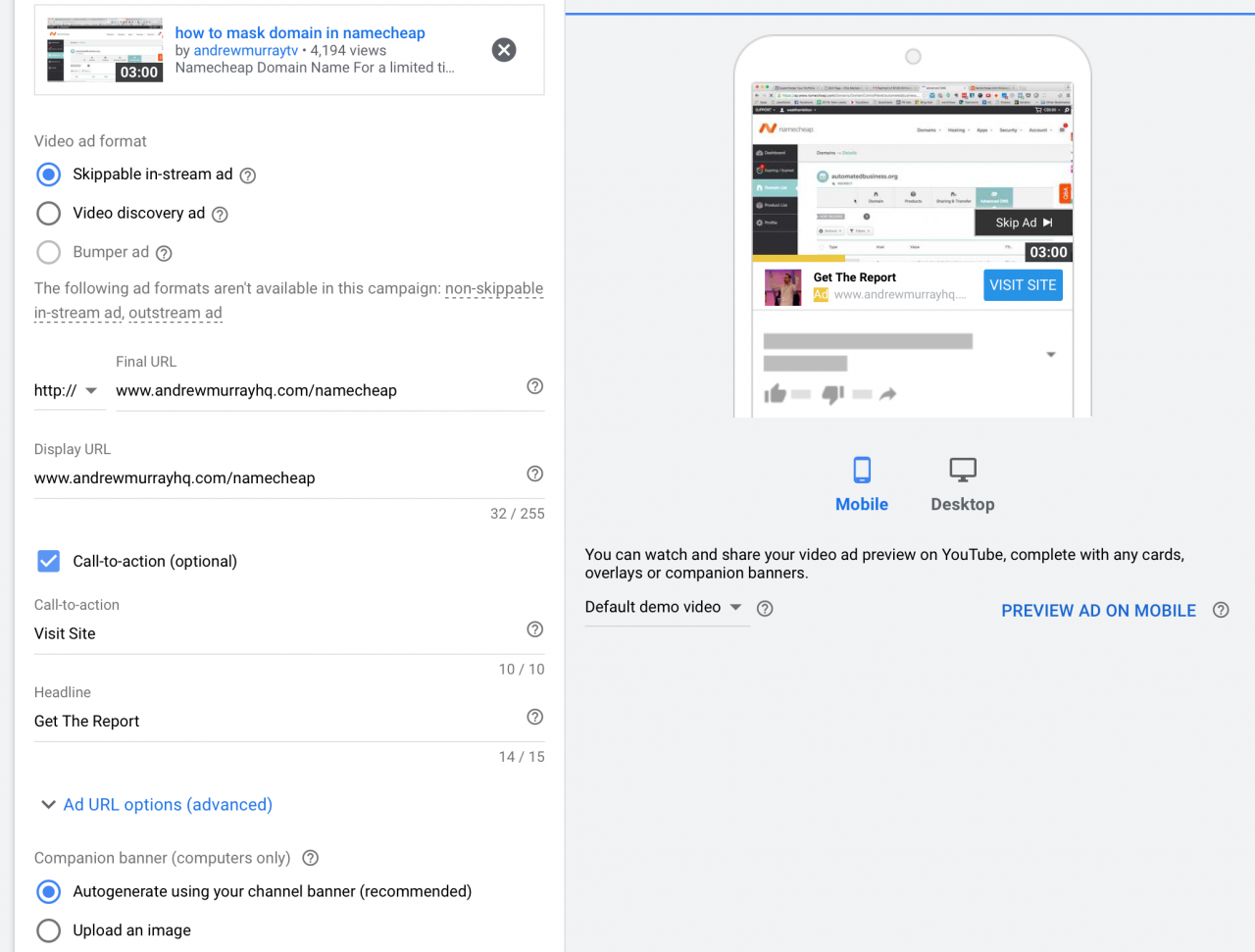The image features a user interface for configuring an online video advertisement. On the left side, there's a white box displaying a thumbnail of a video titled "How to Buy a Domain Name on Namecheap" by Andrew Murray TV, with 1,000 views. This video is 3 minutes long. Below the thumbnail, it indicates that the ad type selected is highlighted in blue.

On the right side, within a gray box, several ad format options are listed from top to bottom: "Skippable In-Stream Ad," "Video Discovery Ad," and "Bumper Ad," with the "Skippable In-Stream Ad" being selected. Below these options, it states that certain ad formats are not available for this campaign, specifically "Non-Skippable In-Stream Ad" and "Out-Stream Ad."

Further down, the "Final URL" is shown as "www.andrewmurrayhq.com/namecheap," which is also mirrored in the "Display URL" field. At the very bottom of the gray box, a message indicates "32 out of 265," next to a blue box with a checkmark that reads "Call to Action."